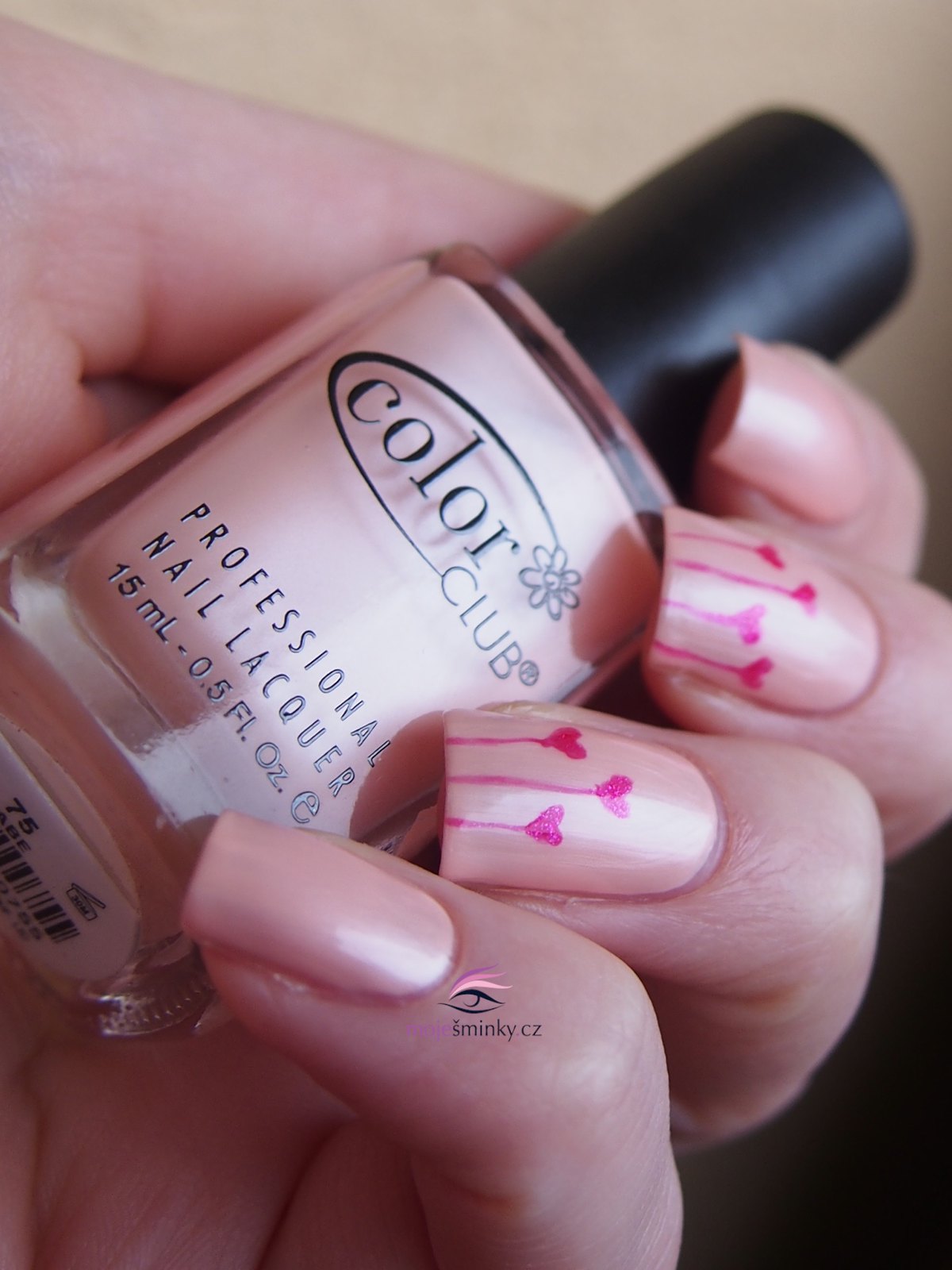In this detailed image, a hand with neatly manicured nails holds a bottle of pale pink nail polish, matching the shade on the nails. The nails are styled with flat, square tops and display a glossy sheen. Two of the nails, specifically the ring and middle fingers, feature intricate designs: hot pink hearts with fine lines emanating from them. The design on one nail has three hearts while the other has four. The nail polish bottle has a black handle and is labeled 'Color Club.' Below the brand name, it states "professional nail lacquer" in bold black letters, and mentions the volume as 15 milliliters (0.5 FL ounces). The overall image highlights the attention to detail in both the nail art and the product design.